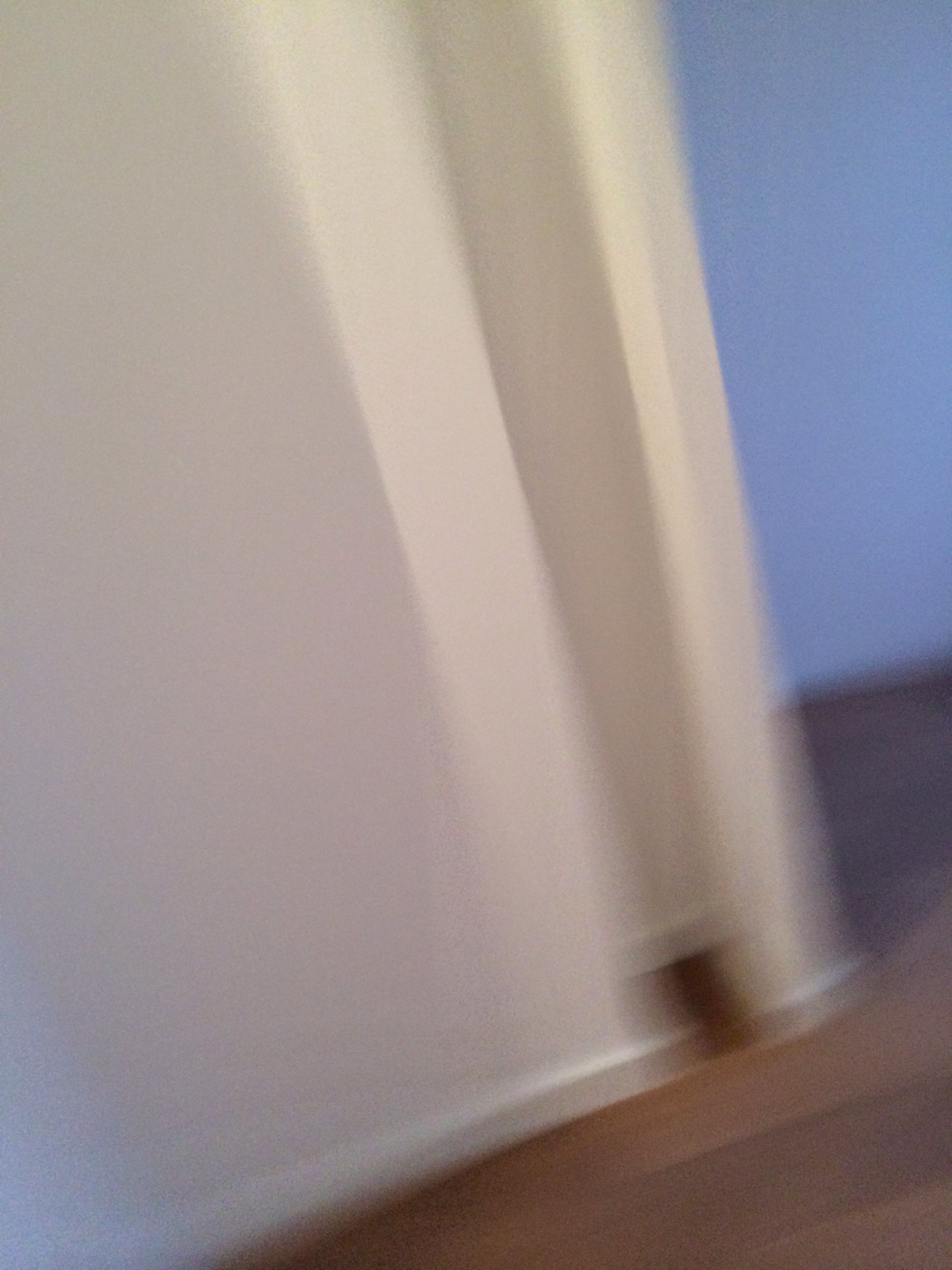This color photograph is an indoor shot characterized by significant blurriness and a slight tilt to the right, creating a leftward tilt in the image. Dominating approximately 80% of the frame, from the top left to almost a triangular space at the bottom right, is a light beige wall. This wall has a vertical indent near the right edge, leading into what seems like a small corridor or enclave. The wall area is well-lit, yet blurry, with a narrow band near its bottom catching the light, which can be seen extending higher up within the indent, casting a slightly darker shadow. In the upper right corner and tapering downward into a triangle, there is a pale blue background that transitions to grey as it moves towards the center right. This hue also appears briefly in the lower left corner. Additionally, the bottom right features a triangle of dark brown, possibly wooden flooring, continuing into the bottom of the white enclave area. The image lacks specific items or text, remaining well-lit but out of focus and grainy, making finer details unrecognizable.